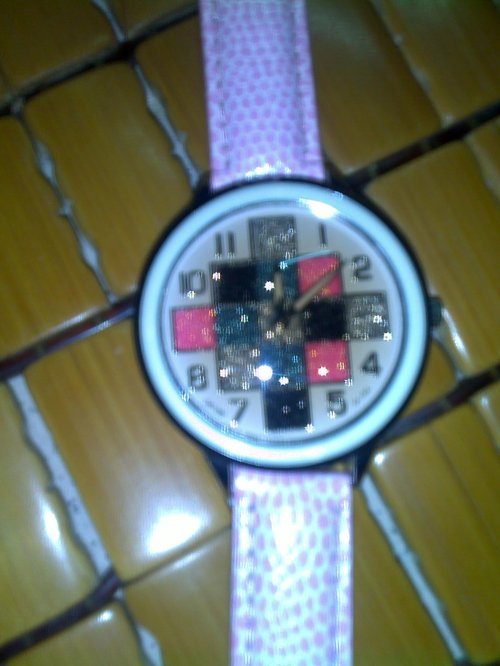A slightly out-of-focus image features a child's wristwatch adorned with vibrant decorations. The watch face displays numbers 1 through 12, interspersed with sparkly sequins and arranged in a square grid pattern. The color scheme predominantly includes gold, pink, and blue, with golden sparkles adding extra flair. The watch hands appear to indicate a time around 12:10. The wristwatch is equipped with white plastic straps decorated with pink and purple polka dots. The background suggests that the watch is either laid on an uneven brown ceramic tile floor or placed on a similarly tiled kitchen table, with a noticeable glare hinting at overhead lighting.